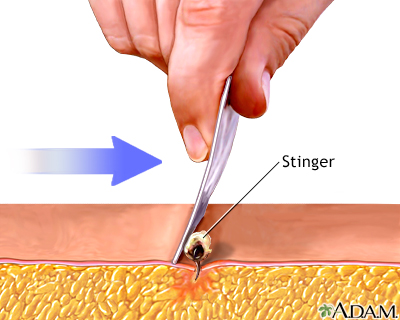The image is a detailed diagram illustrating the process of removing a stinger from the skin. The diagram features a close-up of a person's hand holding a tool, which appears to be a pair of tweezers or a knife. It depicts the upper and lower layers of the skin, with the stinger embedded deep within the lower layer, resembling a small fuzzy object. Arrows and labels direct attention to the stinger and indicate the method to dislodge it. Instead of pulling, the tool is applied in a manner that involves pressing down on the skin to push the stinger out. The bottom layer of the skin is shown as a yellow, corn-like texture, contrasting with the natural skin color of the upper layer. This instructive image is likely from a science book, educating viewers on the anatomy of the skin and the correct technique for stinger removal, despite its somewhat unsettling appearance.